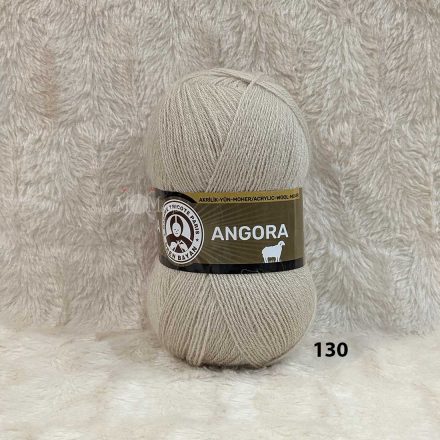The image features a large skein of beige yarn standing upright in the center. The yarn has a light brown hue, slightly darker than the white and beige backdrop upon which it sits, which appears to be a white rug with black lines. This contrast adds visible shadows around the yarn. The background includes a white, shaggy material, possibly a blanket or an article of clothing, textured similarly to the yarn. The label on the yarn is dark brown with white text, prominently displaying "Angora" in white font above a small image of a sheep. Additionally, to the right of the yarn, a circle features an illustration of a person knitting, with surrounding text. Below this circular detail, the numbers "130" are printed in black, possibly indicating the weight or length of the yarn. The overall image exudes a tone of matching earthy and neutral colors, blending the yarn smoothly with its background.